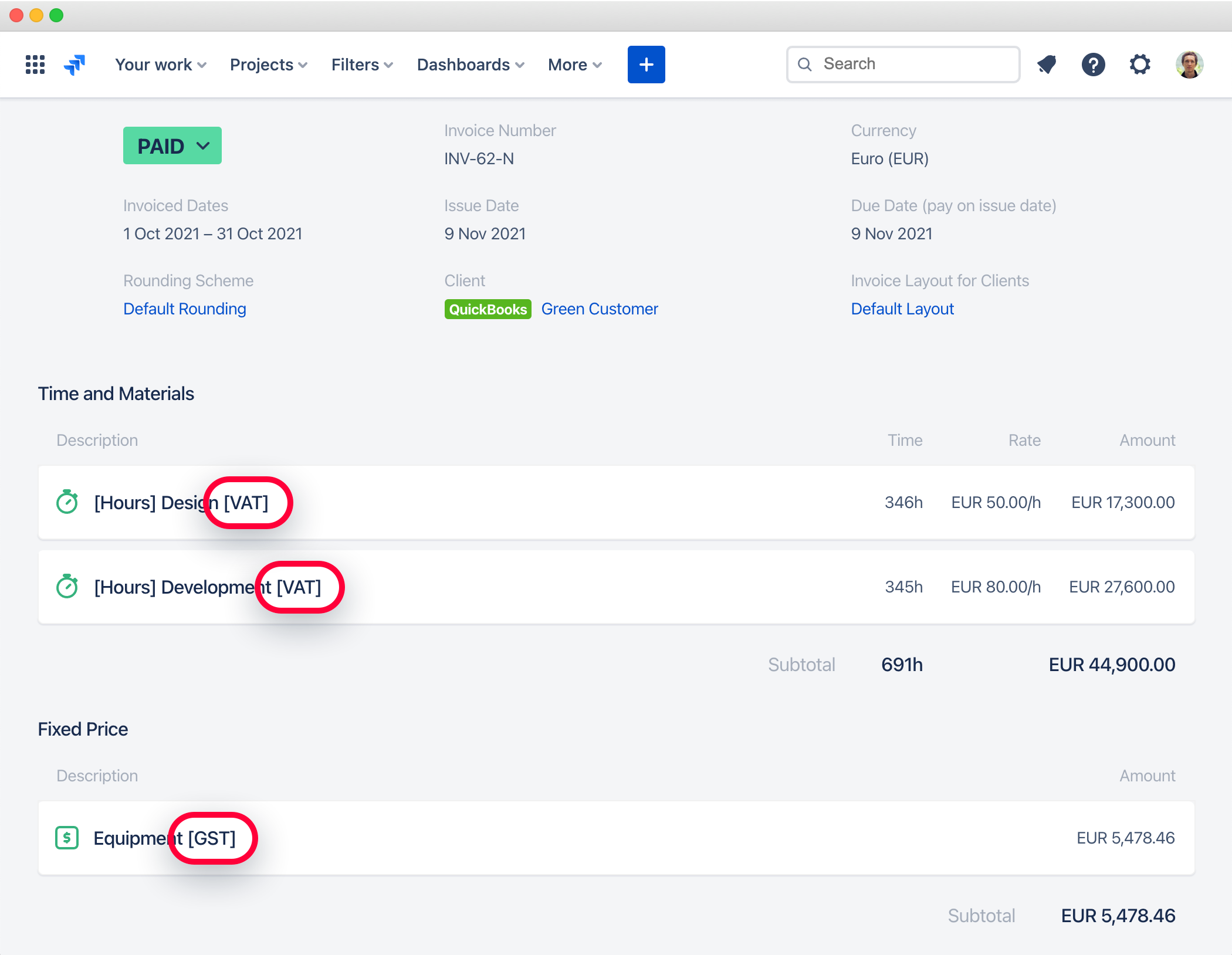**Descriptive Caption:**

The web page displayed in the image appears to be a work-related interface with various navigational elements and detailed information. At the top of the page, the toolbar features several interactive components. On the left, there is an icon consisting of three blue arrows pointing upwards to the right. Adjacent to this are a series of drop-down menu links labeled as follows: "Your Work," "Projects," "Filters," "Dashboards," and "More," followed by a blue button with a plus sign at its center.

To the right of these navigational links, a search box is present, flanked by four icons - a bell, a question mark, a gear, and the user’s profile picture encapsulated in a circular icon.

In the upper left of the main body of the web page, there is a greenish-blue button with the text "Paid," which functions as a drop-down menu. Below this, invoice details are displayed: "Invoice dates: October 1, 2021, to October 31, 2021," "Invoice number: IVN62N," and "Issue date: November 9, 2021."

Towards the middle-bottom section of the page, certain elements are highlighted with circles. The "hours designed" section and "VAT" are circled. Additionally, the "hours development" section is noted with "VAT" circled, and under the "fixed price" category, "GST" next to "equipment" is highlighted.

In the bottom right corner of the page, the subtotal is listed as "Euros 5,478.46."